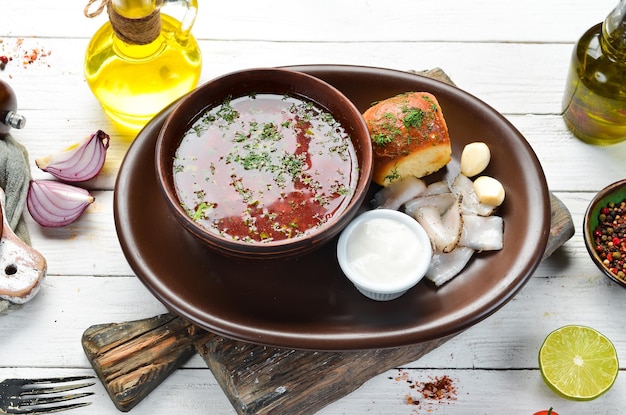This color photograph in landscape orientation captures an overhead view of a meal artfully arranged on a white or pale wooden table. The main focus is a deep, oblong brown platter made of a shiny, ceramic material, resting on a dark brown, weathered serving board with a striking fishtail design on the left. Inside the platter, a large, round brown bowl holds a milky pink soup garnished with brown spices and finely chopped green herbs, possibly chives or parsley. To the right of the bowl, a square dinner roll with a green herb on top sits beside two whole garlic cloves and a ramekin of white dipping sauce. Additional items surrounding the platter include a green lime half, slices of red onion, and a container likely holding olive oil, partially cut off at the edge of the frame, all contributing to a representation of detailed and realistic food photography.